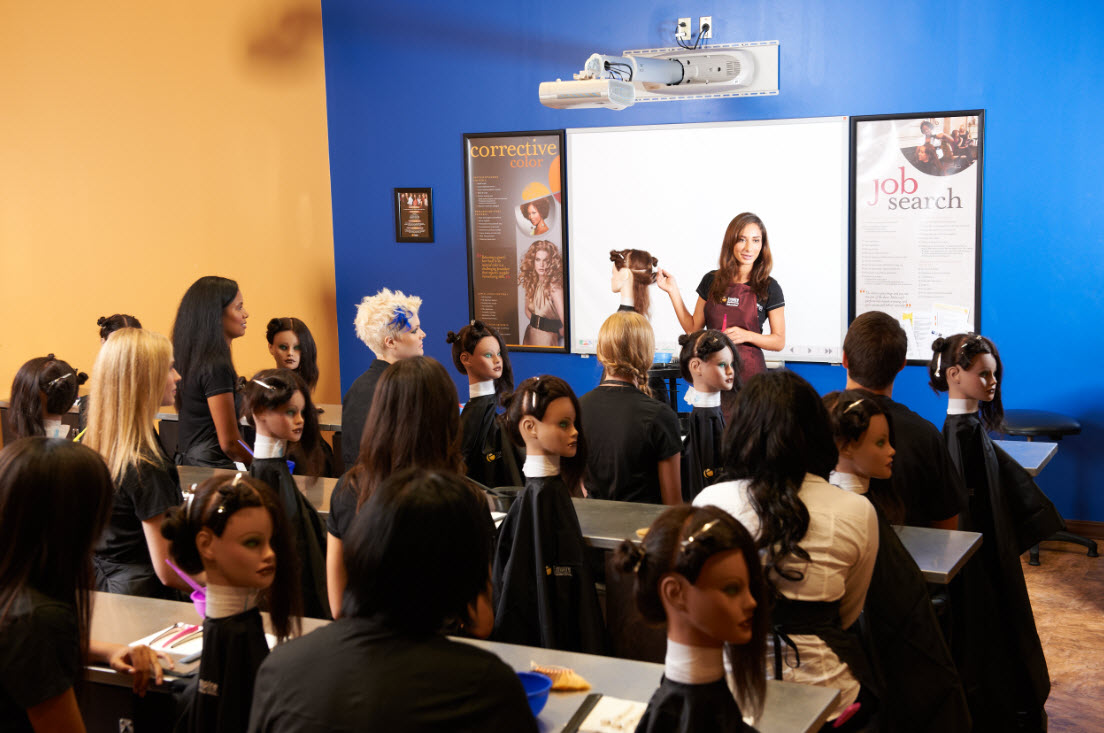This detailed photograph captures a bustling classroom scene in a cosmetology class, focusing on hairdressing techniques. The room is organized with three rows of long metal tables, each occupied by students working on mannequin heads. The image is taken from the back, showcasing the student’s back and their long hairstyles, primarily brunettes, with the occasional blonde and a male student with short hair sitting in the front row. Each mannequin features a hairstyle with the right side pinned up and short, while the left side's hair cascades nearly to the table. The instructor, a Caucasian woman with long brown hair, stands at the center front of the room, wearing a black polo and a red apron, gesturing towards her mannequin that mirrors the students' practice heads. She holds a pink comb in her left hand.

The setting features a prominently blue back wall with a whiteboard behind the teacher. The whiteboard bears no writing but is flanked by distinct posters. On the left, an informational poster on corrective hair coloring features an African-American woman with natural hair above another woman with curly brown hair, adorned with white, goldish-yellow, and orange text. On the right, another poster reads "JOB" in red letters and "SEARCH" in black below, with additional text that is indiscernible from the photograph’s perspective.

The classroom's left wall is a pale orange, integrating with the vibrant learning environment. Above the whiteboard, a projector is mounted, ready for instructional use, connected to visible electrified receptacles. This meticulous setup along with the mannequin heads and styling tools on the tables emphasizes a hands-on learning experience pivotal for mastering the art of hairdressing.